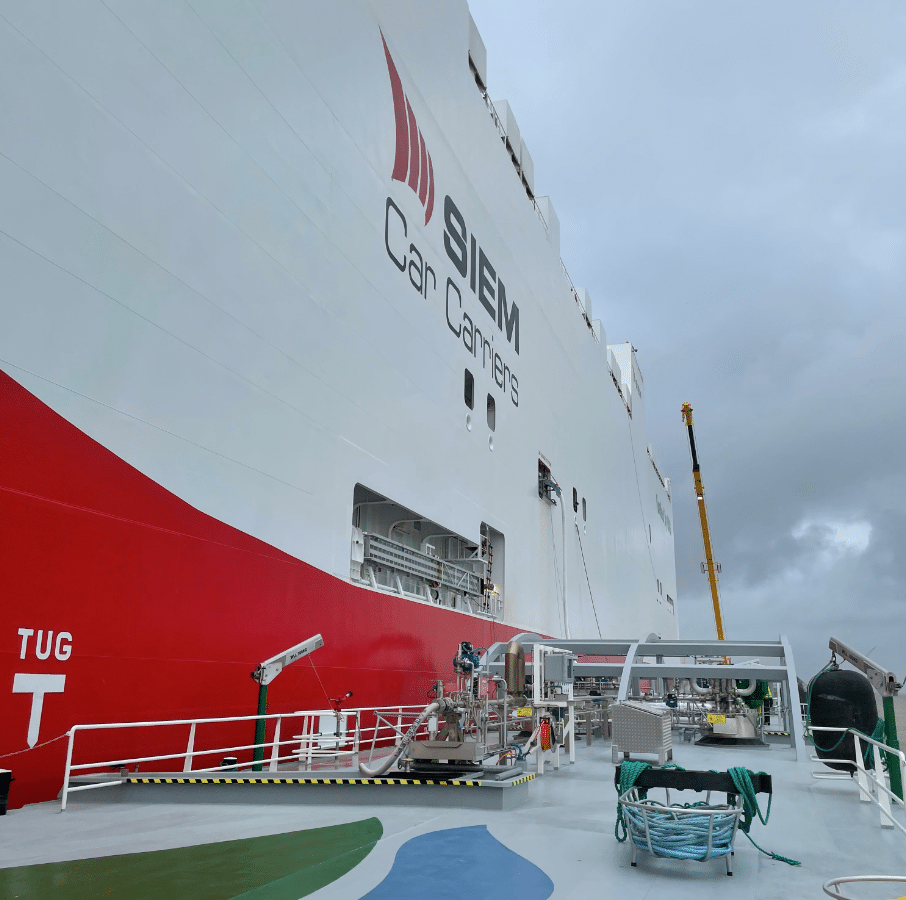This photograph captures the side view of a colossal white and red cargo ship named "SIEM Car Carriers." The ship is painted predominantly white with a red base and features a logo with four vertically aligned red stripes resembling sails. The name "SIEM Car Carriers" is prominently displayed in white text on a red background on the side of the vessel. The scene is set on a cloudy day with a gray sky, adding a dramatic backdrop to the ship's clean, imposing structure. The vessel sits docked, with visible contact points against the dock. The foreground displays a cluttered dock area featuring a fenced deck, coiled hoses, and various equipment such as cables, life jackets, life rings, and metal containers. A large, yellow crane looms over the ship, indicating ongoing activity, although no personnel are visible in the scene.